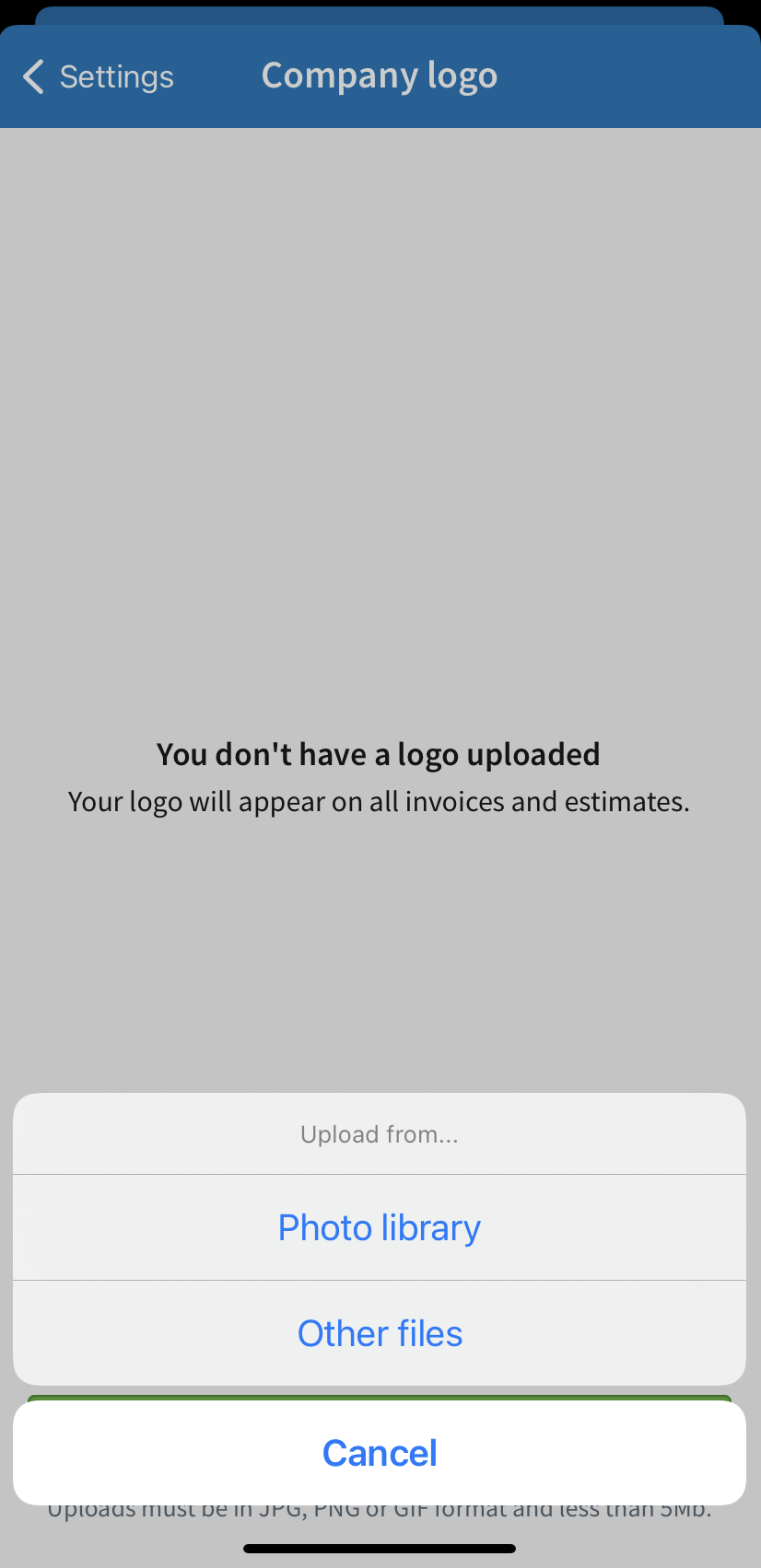The image displays a smartphone screen with the app's company logo settings page open. At the top, a black rectangular bar is overlaid by a blue rectangle labeled 'Settings' with a left-pointing arrow. Beside the arrow, 'Company Logo' is clearly displayed.

The center of the screen is primarily a blank, gray background. In the middle, the text reads, "You don't have a logo uploaded." Beneath this, a message states, "Your logo will appear on all invoices and estimates." Further down, a gray rectangular box invites the user to upload a logo, presented with the text "Upload from..." and three blue clickable options: "Photo Library," "Other Files," and "Cancel".

At the very bottom, the cancel button slightly overlaps some small print, with a thin black line accentuating the screen's edge.